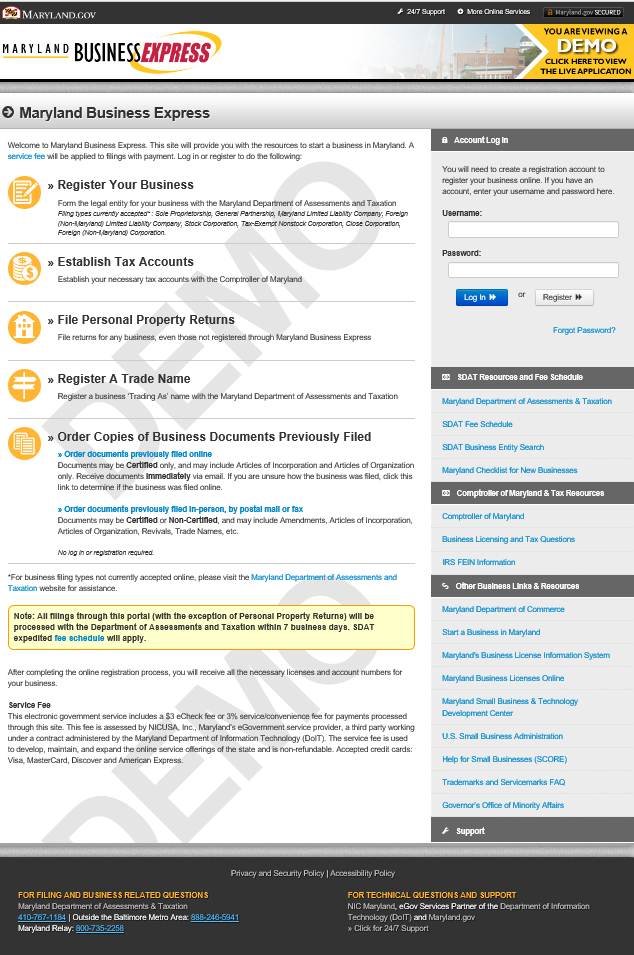The image depicts a webpage with a structured and professional layout designed for business-related services. At the very top, a sleek black banner features the site name "Maryland.com" in prominent white letters, creating a striking contrast. Directly beneath this, another banner reads "Maryland Business Express," suggesting a focus on facilitating business transactions and activities. Adjacent to this banner, a notification indicates that the viewer is currently navigating a demo version of the site, with an actionable link inviting users to "Click here to view the live application."

The main body of the webpage has a predominantly white background, providing a clean and uncluttered look. The content is presented in black text and is organized into a series of action-oriented navigation tools. These include essential business services such as "Register Your Business," "Establish Tax Accounts," "File Personal Property Returns," "Register a Trade Name," and "Order Copies of a Business Document," each serving as a gateway to more detailed processes and forms.

On the right side of the page, there is a vertically-aligned gray sidebar that further enhances user navigation. This sidebar includes additional resources such as "Login Instructions" and other pertinent links, aimed at guiding users through the website's various functionalities. The overall design is functional and user-friendly, geared towards providing comprehensive support for Maryland-based businesses.